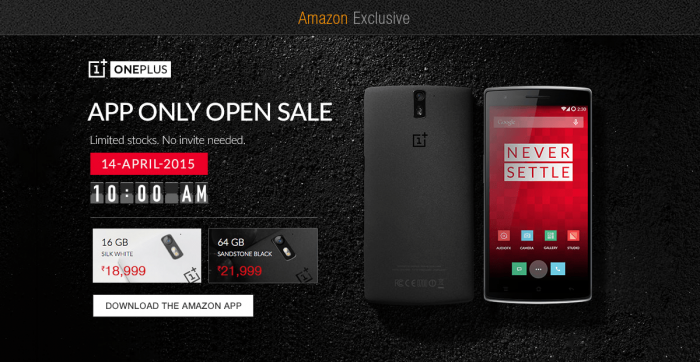Taken in portrait mode, the image showcases an announcement for a OnePlus cellphone, detailing its release specifics on an Amazon-exclusive sale. Across the top of the image, a sleek, long black rectangle contains the text "Amazon Exclusive" with "Amazon" in a bold orange and "exclusive" in gray. 

Beneath this header, a white box prominently displays the OnePlus logo, featuring a '1' in an actual number form housed within a black square. Further details appear below in white text, indicating an "app-only open sale" with "limited stocks" and "no invite needed." 

A striking red rectangle gives the sale date as "14-April-2015." Just below this, in large, digital alarm clock-like numbers, the time "10:00 AM" is displayed. 

Centering the image, a smartphone takes the focal point, branded with the bold slogan "Never Settle" in red on its screen.